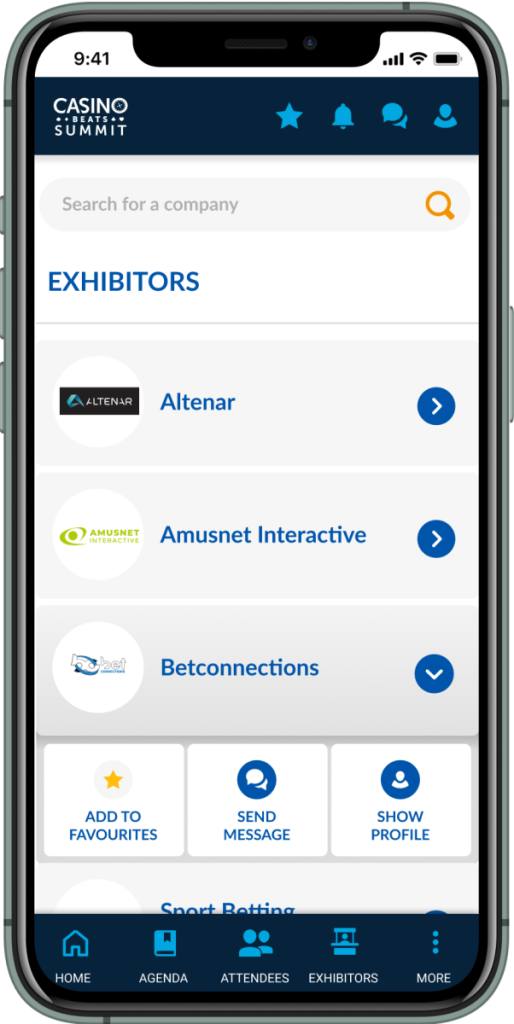The image showcases the user interface of a mobile device with full cellular service bars, Wi-Fi signal, and battery status visible at the top. In the background, a casino-themed event is apparent with several interactive icons and features displayed.

- **Top Navigation Bar**: Shows network indicators—full signal bars, Wi-Fi icon, and fully charged battery.

- **Event Apps and Icons**:
  - **Casino reminder**
  - **Beats (possibly audio or music streaming)**
  - **Summit, Star, and Bell (likely event reminders or favorite tags)**
  - **Chat feature icon, depicting a speech bubble** 

- **Search Function**: 
  - An orange magnifying glass symbol for searching companies and exhibitors.
  - The options to "Add to Favorites" and "Send Message" with associated icons: a gold star and a chat bubble, respectively.

- **Exhibitor Logos**: 
  - “All Tenor” highlighted with a black logo.
  - "AmuseNet Interactive" featuring a green logo with a blue circle and white arrow pointing right.

- **Menu and Features**:
  - Beck Connections enlisted with a blue circle/white arrow and a gold star underneath.
  - Show Profile option depicted by a silhouette icon.
  - A horizontal navigation menu at the bottom includes:
    - **Home** with a house icon.
    - **Agenda** symbolized by an open book.
    - **Attendees** represented by two human silhouettes.
    - **Exhibitors** shown as a stand with a figure inside.
    - **More** depicted by three blue dots. 

The phone hardware details are also visible:
- Volumes keys and camera button on the left side.
- Power key on the right.
- At the top, the speaker and front-facing camera are noticeable.
- The phone frame has a sleek, gray-silver finish.